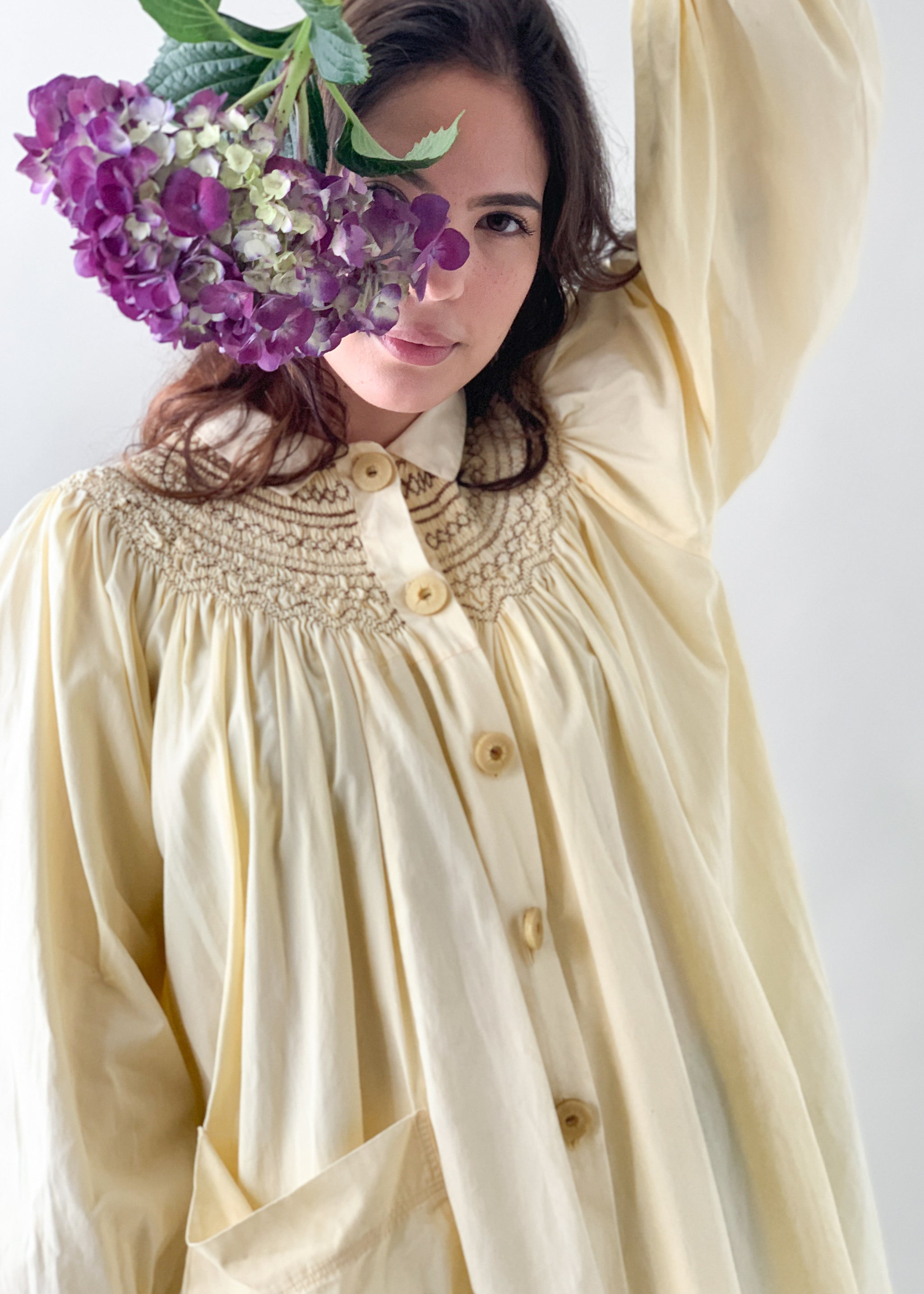The image is a professionally taken photograph of a young Caucasian woman against a solid white background. She is dressed in a vintage-style, oversized smock that is a sort of off-white or beige color, heavily wrinkled with a loose fit. The smock features large round buttons running down the front and a substantial pocket on the left side (viewer's right). There is intricate embroidery and smocking around the collar, which adds a touch of detail to the garment.

The woman has long, dark brown hair cascading past her shoulders, fair skin, and expressive brown eyes. Holding her left arm aloft, she clutches a sizeable bouquet of flowers that obscures her eye and part of her face. This bouquet, composed of small purple violets and white flowers with green stems and leaves, hangs upside down and almost matches the size of her head. Her lips form a bemused expression as she gazes directly into the camera, giving the photograph an intimate and whimsical feel.